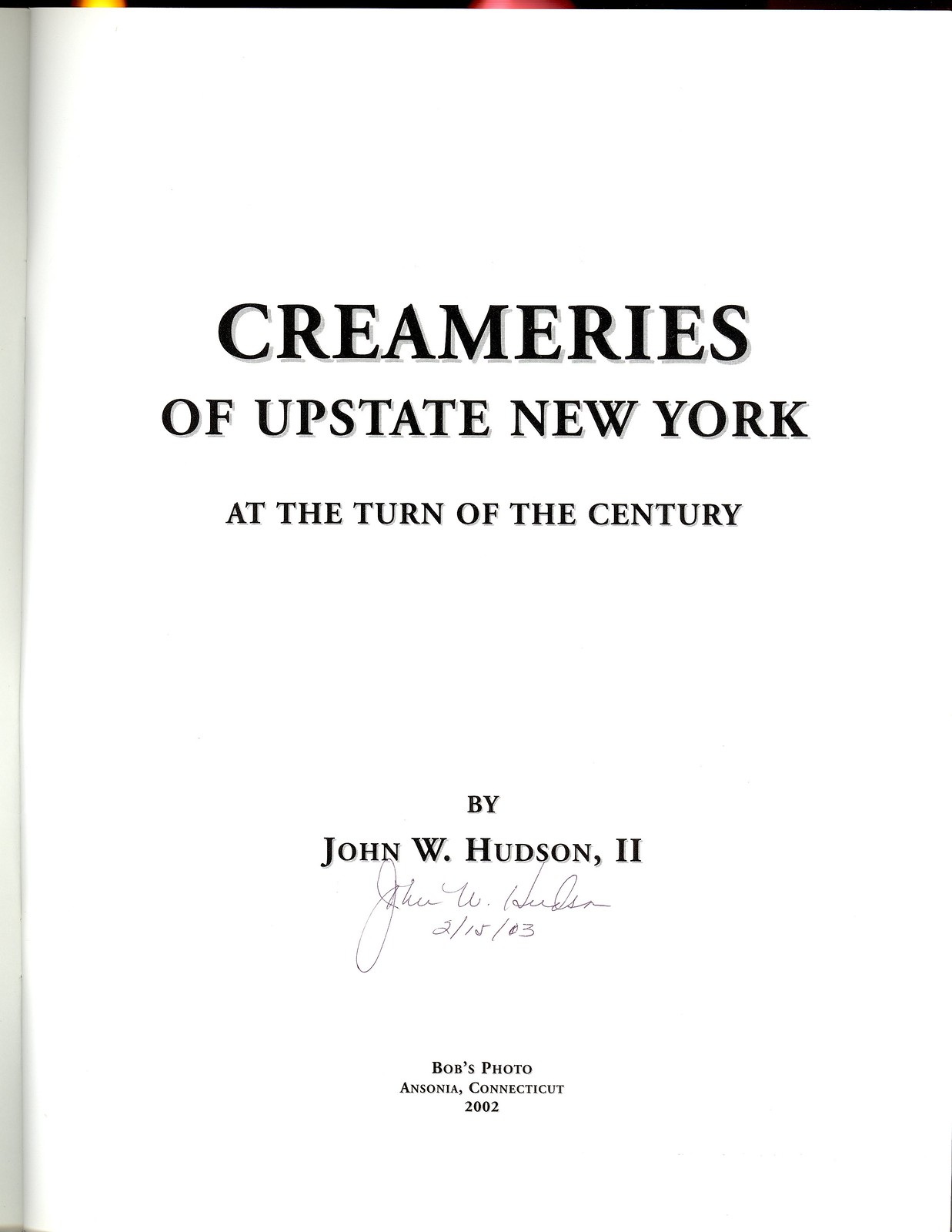The image exhibits the title page of a book, showcasing a very high-quality scan or photograph. The book, titled in bold, black font, reads "Creamers of Upstate New York at the Turn of the Century" by John W. Hudson II. Directly beneath the author's name lies his signature, "John W. Hudson," penned in cursive with a date next to it, "2-12-03" or "2-15-03." Additionally, the page credits "Bob's Photo, Ansonia, Connecticut, 2002." The page is white with no other visible details against a flat, white background. Some darker, possibly black, regions with yellow and a red bar might be observable beyond the page's edges, hinting at the surrounding space.